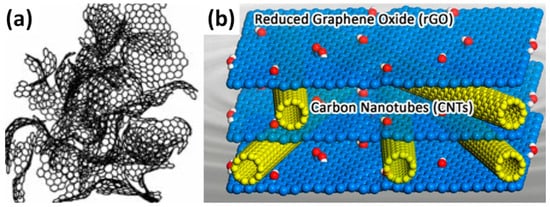The image is a side-by-side comparison of two labeled photographs, A and B. Photo A, on the left, displays a white background with a crumpled, honeycomb-like structure made of white, paper-thin material with gray-black edges. Photo B, on the right, exhibits a detailed illustration of Reduced Graphene Oxide (RGO) and Carbon Nanotubes (CNTs). It features a gray background with layers of blue sheets representing graphene oxide, interspersed with green, bumpy tubes (CNTs), and red and white atoms scattered across the layers. The layers and atoms are depicted with labeled elements, illustrating the complex structure of RGO and CNTs on a blue tray.